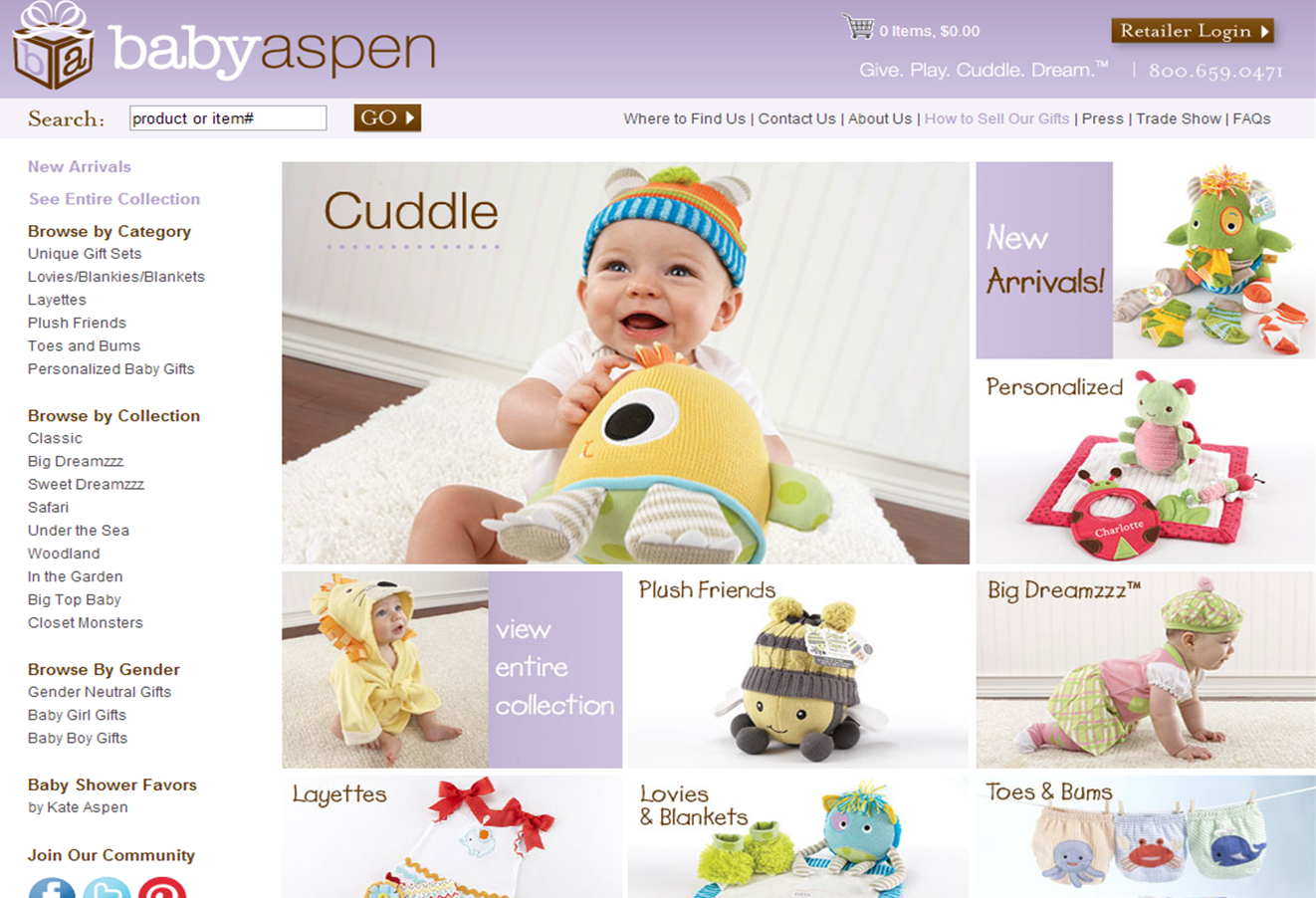The screenshot showcases the Baby Aspen website, dedicated to offering an array of baby gifts and items. The top-left corner features a child's toy, accompanied by the brand name "Baby Aspen" to the right, with "Baby" in white and "Aspen" in brown lettering. Adjacent to this, there is a shopping cart icon displaying the total price of selected items and a retailer login option in the top-right corner. The website's tagline, "Give Play Cuddle Dream," is prominently displayed alongside a contact number, 800-659-0471.

A central image showcases an adorable baby holding a toy, surrounded by a selection of clickable sections, each highlighting different product categories. These include "New Arrivals," "Personalized," and "Big Dreams." To the left, there is a section titled "Plush Dreams," referring to stuffed animals. Another clickable square offers the option to "View Entire Collection."

Additional product categories include "Layettes," "Lovies and Blankets," and "Toes and Bums," hinting at handmade clothing and toys. The user can navigate the site via a sidebar on the left, allowing browsing by category, collection, gender, and baby shower favors. Social media icons for Facebook and potentially Twitter (though partially visible) encourage users to join the Baby Aspen community.